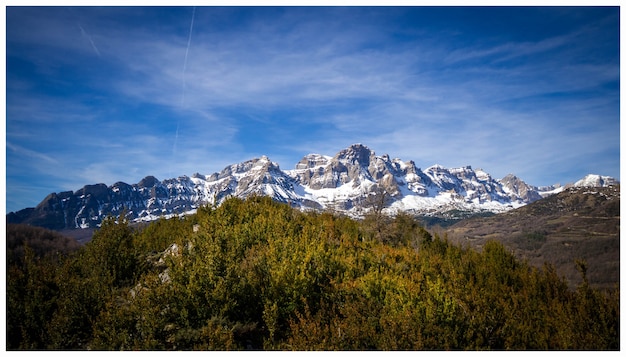This is a horizontal, aerial photograph capturing a breathtaking mountain landscape. In the background stretches a majestic mountain range with prominent, rocky cliffs adorned with patches of snow, suggesting early fall with some areas where the snow has partially melted. The peaks rise against a backdrop of a deep blue sky scattered with thin white clouds and identifiable jet streams from recent flights. In the foreground, lush green trees blanket the hills, so dense that the ground beneath them is obscured, though patches of dirt and the occasional glimpse of snow are visible. The mid-ground features rolling, grassy hills interspersed with trails or roads, and dotted with bushes and smaller trees in varying shades of green and brown. This sunlit scene encapsulates the serene beauty of nature, with the crispness of the air almost palpable through the image.